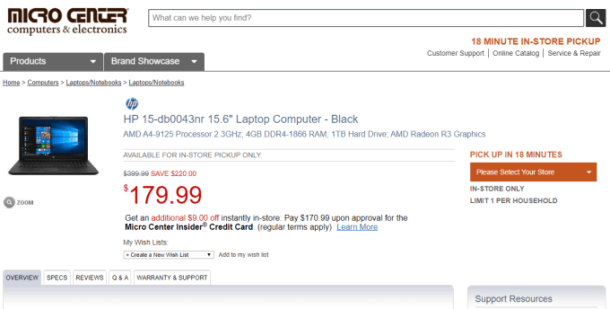This image is a detailed screenshot of the Micro Center Computers and Electronics website homepage. Dominating the top portion is a prominently displayed, long rectangular search bar with a placeholder text that reads, "What can we help you find?" followed by a magnifying glass icon for initiating searches.

Below the search bar, there are two main navigation tabs: one labeled "Products" and the other "Brand Showcase." To the immediate right, highlighted options include an "18-Minute In-Store Pickup" service, "Customer Support," "Online Catalog," and "Service and Repair."

Featured prominently on the page is a specific product listing for the **HP 15-DB0043NR 15.6" Laptop Computer in Black**. Detailed specifications are provided: 

- Processor: AMD A4-9125, 2.3GHz
- Memory: 4GB DDR4-1866 RAM
- Storage: 1TB Hard Drive
- Graphics: AMD Radeon R3

The product is available exclusively for in-store pickup at a discounted price of \$179, down from the regular price of \$399.99. An additional offer allows customers to save \$9 instantly in-store, reducing the price to \$170.99 if they are approved for the Micro Center Insider credit card, subject to regular terms and conditions. This deal is limited to one per household.

Additional options for the product include adding it to a wishlist, selecting a store for the 18-minute pickup, and several informational tabs such as Overview, Specs, Reviews, Q&A, Warranty, and Support. Support resources are also available to address any queries.